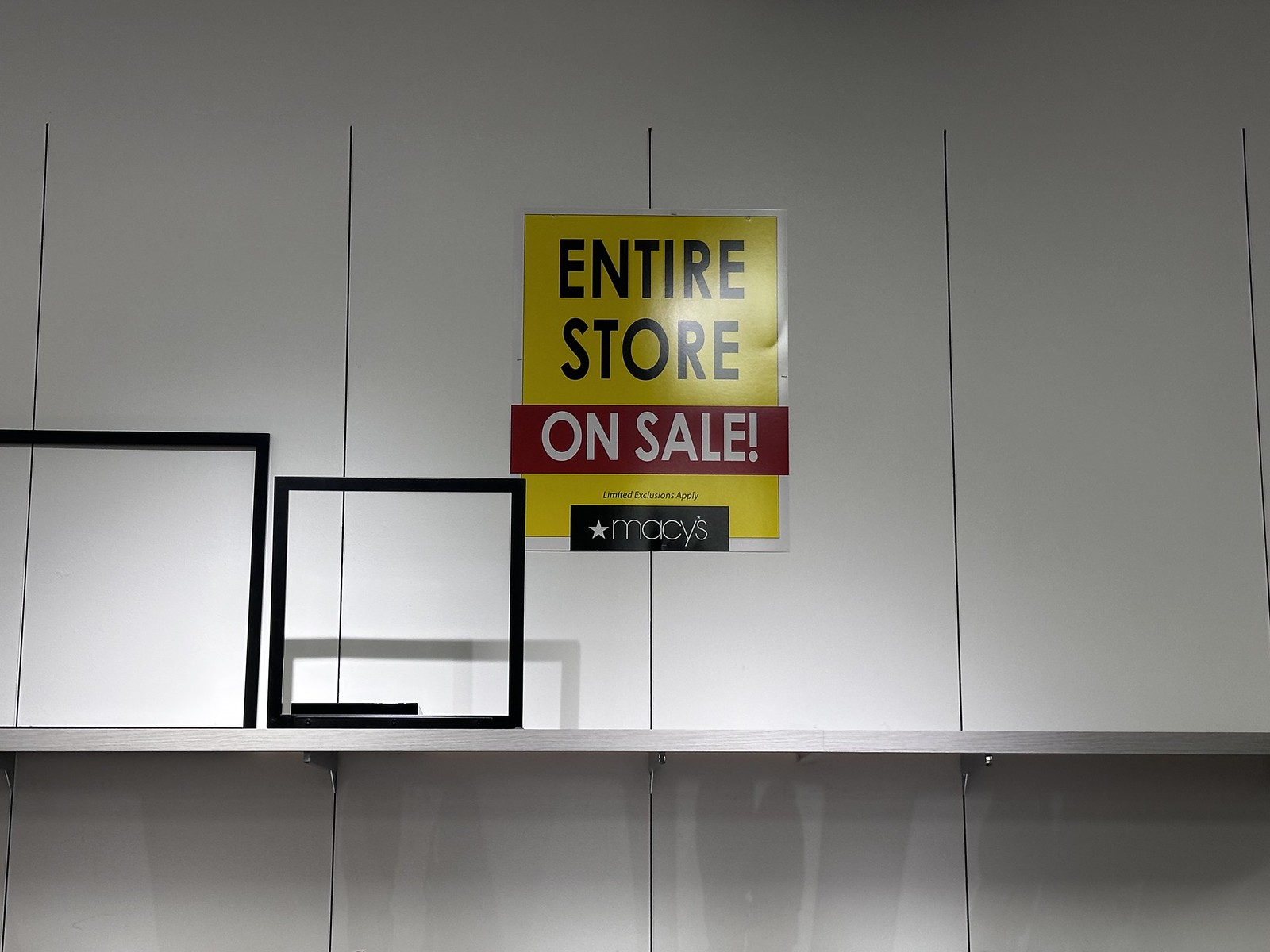This square-shaped image showcases a neatly hung poster on a white wall, centered within the frame. The poster also follows a square format and is adorned with a clean white border. The upper section of the poster is dominated by a bright yellow background with the bold black text "ENTIRE STORE" prominently displayed. Just below, a vibrant red strip hosts the words "ON SALE!" in striking white letters. The lowest portion states "Limited exclusions apply" in smaller text. Adjacent to this text is a simple yet impactful artwork of a white star. Beside the star is the recognizable "Macy's" brand name. The white wall behind the poster features five evenly spaced black lines running horizontally. To the left of the poster, there is a partially visible object whose details are unclear.